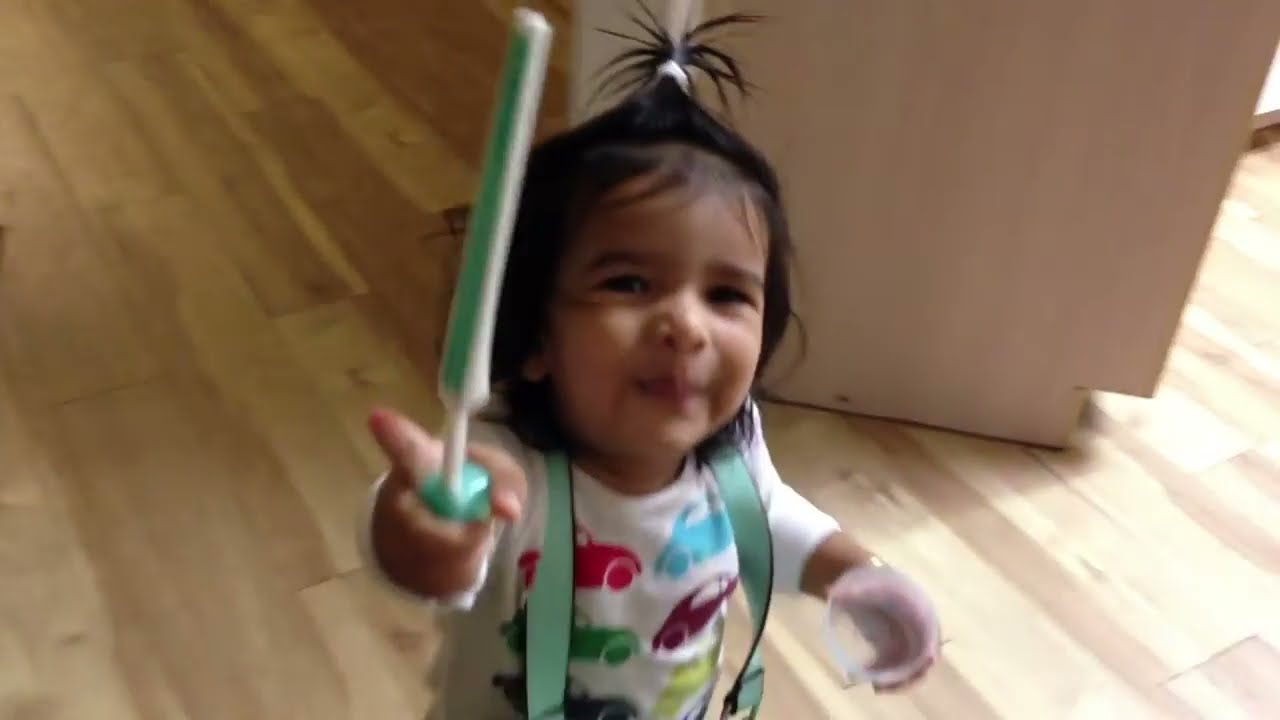The horizontally aligned rectangular picture captures a close-up of a small girl with slightly blurry focus. Centered in the image, the girl is smiling with her mouth closed, revealing her brown eyes and slightly dark skin. Her dark black hair is pulled up into a short ponytail on top of her head, secured with a white tie. She wears a white long-sleeved shirt adorned with colorful cars in various hues—red, blue, green, purple, and yellow. The girl holds a clear plastic cup in her left hand and displays a green and white toothbrush in her right hand, directed towards the person taking the photograph. Teal-colored suspenders with black stripes run over her shoulders, hinting at a small backpack she might be wearing. She stands on a light brown wooden tiled floor, with a matching light brown cabinet visible behind her, suggesting the setting is a kitchen. The photograph is taken from an above-down angle, accentuating the floor and background details.